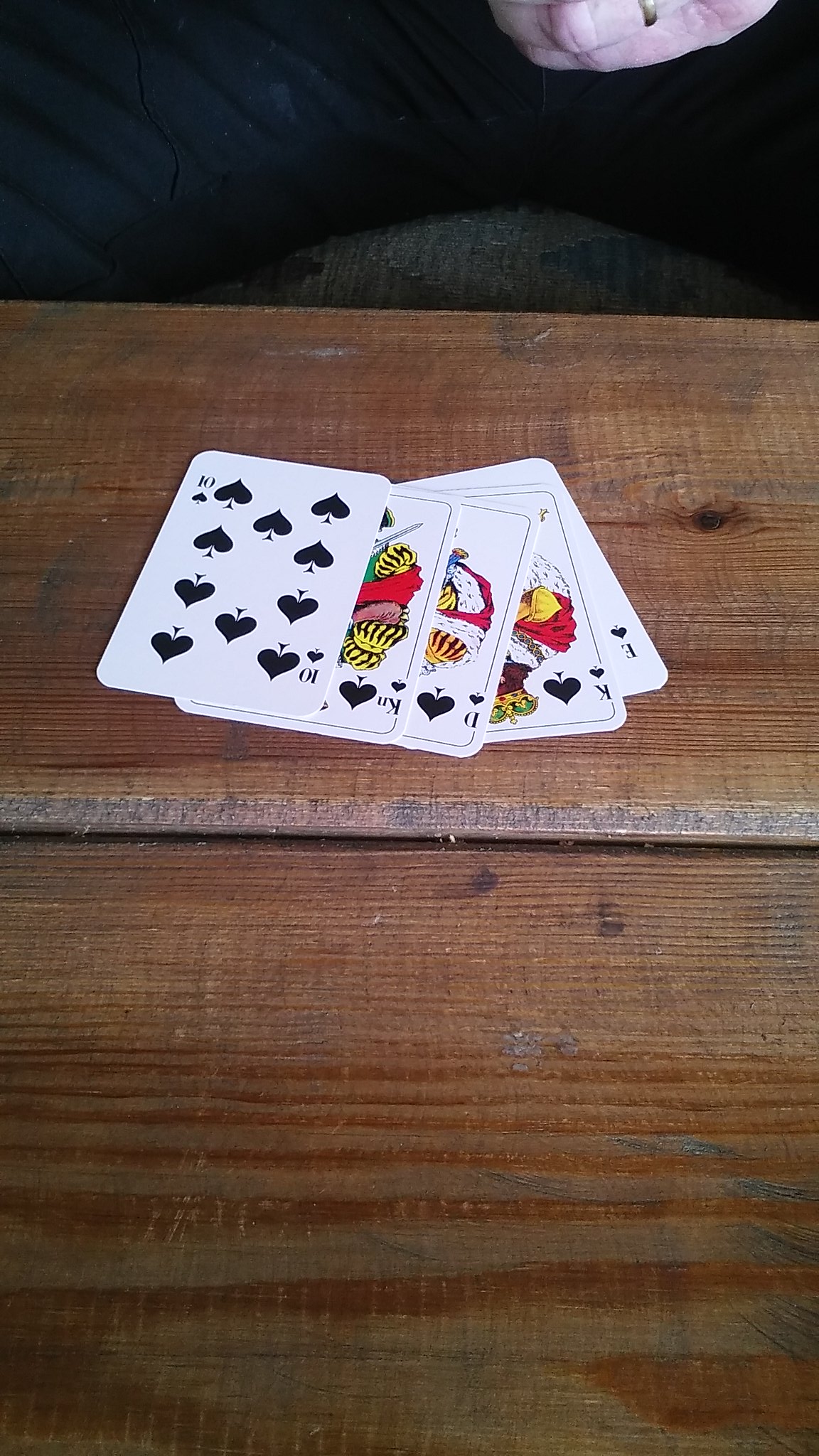On a very worn pine coffee table, featuring several scratches, cigarette burns, and small bits of chips lodged in its cracks, lie five standard rectangular playing cards. The table, neglected and beaten up, serves as a testament to its heavy use. 

In the northern position of the scene, a person wearing black slacks is seated on a low couch or chair that is gray with blue accents.

The playing cards displayed on the table include:
1. Ten of spades.
2. King of spades – adorned with yellow, pink, and red frills.
3. Jack of spades – featuring an orange outfit, a red cape, and a white, fluffy underlayment.
4. Another king of spades – distinguished by a green crown with gold accents, brown hair, and a red cape with a white frilly underlayer.
5. A partially visible spade card, details of which remain indistinguishable.

This image captures a moment of quiet reflection or perhaps a paused game, set against the backdrop of a table that has clearly seen better days.